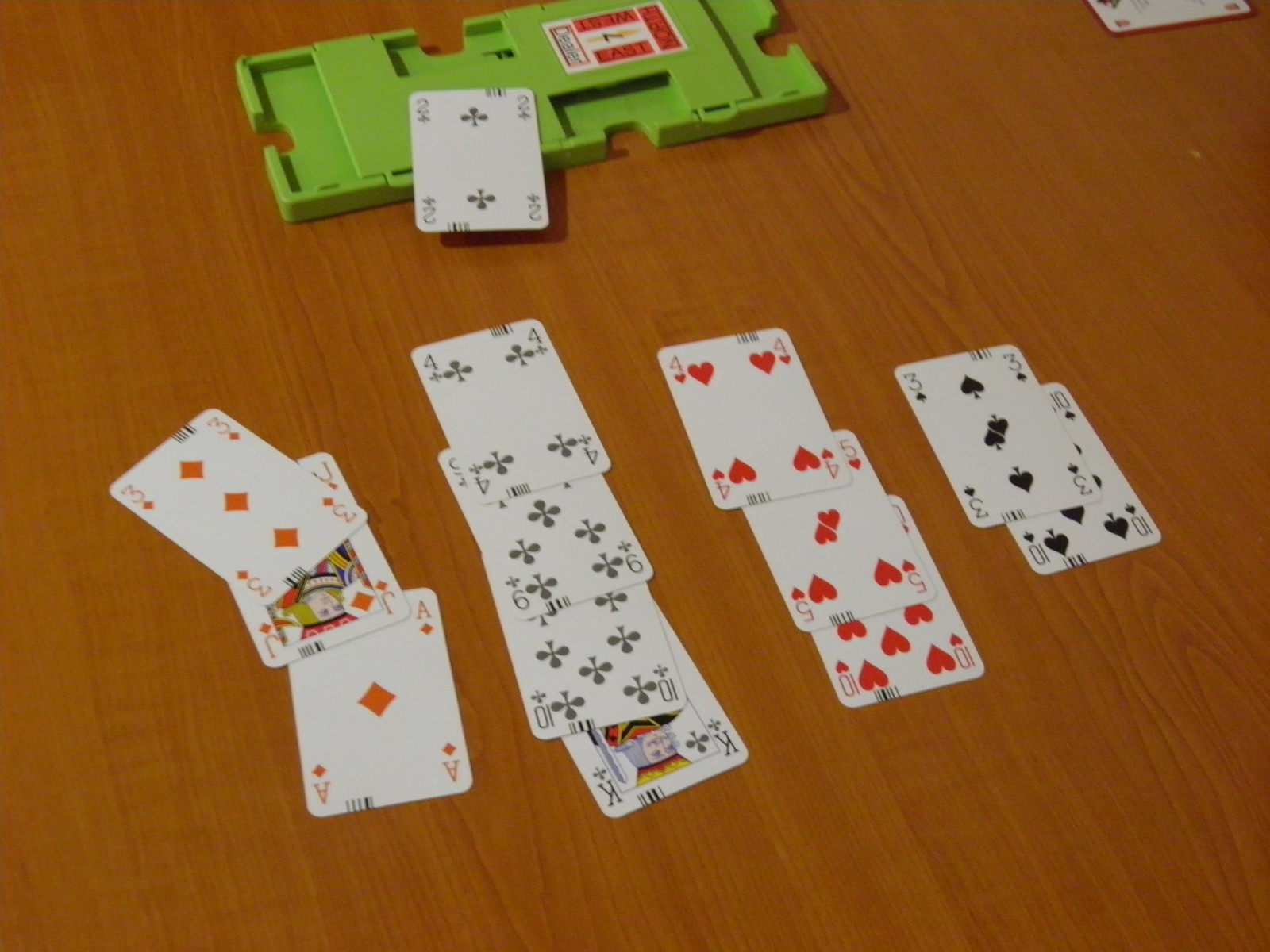The image captures a wooden table with a realistic wood grain effect, spread with an assortment of playing cards in a methodical layout. The cards are arranged in four distinct columns, organized by suits. From left to right:

- **Diamonds:** This column includes the top three cards clearly visible, starting with three of diamonds, followed by the half-hidden jack of diamonds, and finishing with the ace of diamonds.
- **Clubs:** Displayed from top to bottom, the club suit includes the four of clubs, nine of clubs, ten of clubs, and king of clubs. The cards are staggered slightly downward, allowing each card's face to be mostly visible.
- **Hearts:** The column of hearts has a straightforward arrangement with the four of hearts on top, followed by the five of hearts and the ten of hearts.
- **Spades:** The final column features only two cards: the three of spades at the top and the ten of spades below it.

At the very top of the image rests a green plastic object, roughly rectangular in shape with strategically cut-out sections. This might be used as a cardholder or dealer device. Embedded within this green structure is a smaller card or rectangle highlighted by red rectangles around its edge and displaying a number seven in the center. Additionally, the two of clubs is seen partially resting on this green object.

Overall, the scene presents a neat and organized display of playing cards on a wooden table, complemented by a mysterious green plastic object that adds an element of intrigue.